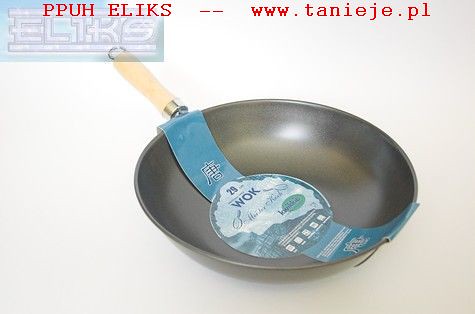The image depicts a professional product photo of a new, nonstick wok set against a subtly varied tan background that transitions to a slightly darker shade on the lower right. At the top of the image, the red text "PPUH ELIKS -- www.tanieje.pl" is prominently displayed. In the upper left-hand corner, there is a semi-transparent, faint blue rectangle containing the word "ELIKS" framed by white bars at the top and bottom with darker blue edges. The central focus is on the wok, which has a light wood handle with a silver semicircle at the end and a silver connector. The main body of the wok is a silver-gray color, signifying a smooth, nonstick surface. Attached to the wok is a teal and white paper tag featuring a central circle that reads "wok" along with other smaller, unreadable details. The tag also includes Asian characters and a design resembling a building, split into a dark blue and white half-circle, adding an extra layer of visual detail to the product's presentation.